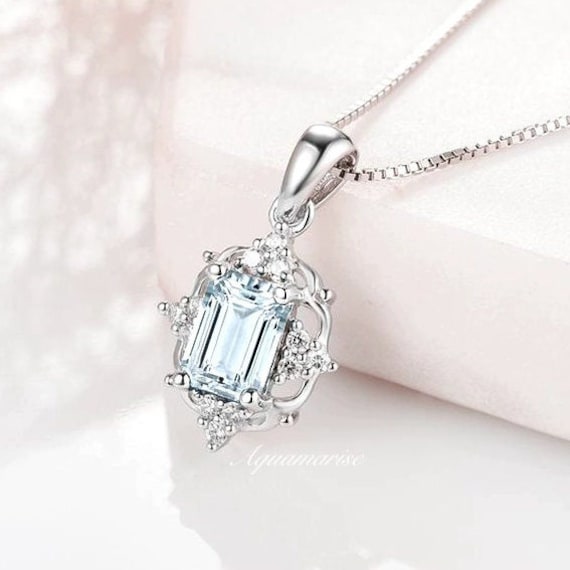The image showcases a close-up view of a silver necklace with a pendant that prominently features a light blue, square-shaped gemstone, possibly aquamarine. The gemstone is surrounded by smaller white diamonds, with three diamonds positioned equidistantly on the top, left, right, and bottom sides of the blue gem. Each diamond setting comprises three small silver beads. The pendant itself is framed by a larger silver square, embellished with silver beads at the corners to securely hold the square gemstone in place. The necklace chain is partially visible, and the entire piece is elegantly displayed, hanging off a white box positioned in the upper right corner of the frame. This box rests on a reflective, shiny white table, casting soft shadows. On the box beneath the pendant, the word "aquamarine" is inscribed in white script, subtly blending with the white surface. The necklace, resting on a pink box, highlights its intricate details against a pristine backdrop.